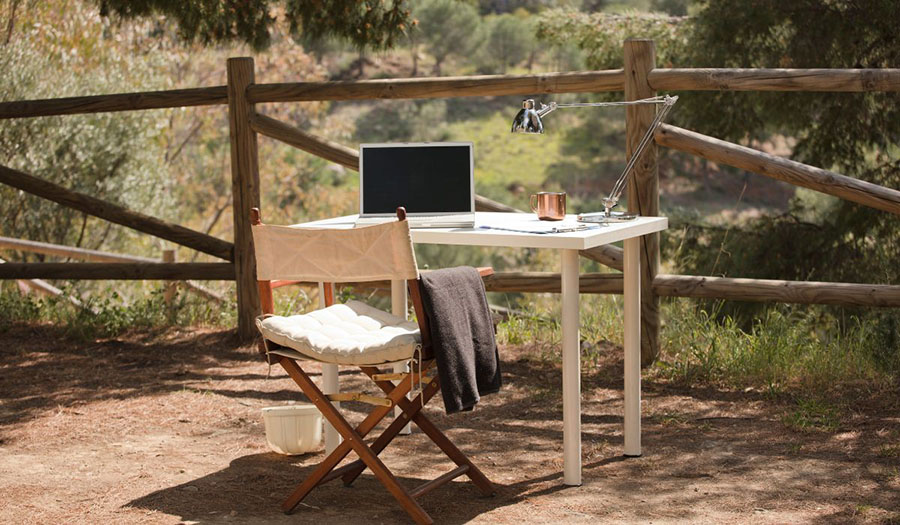This serene and picturesque outdoor photograph, taken in a horizontal rectangle format, captures a tranquil scene set deep in the woods. The backdrop features a dense array of trees and bushes, alongside a rustic handmade wooden split-rail fence that runs across the frame. In front of this charming natural boundary is an unexpectedly modern and minimalist workspace. A sleek white desk, reminiscent of IKEA design, is central to the image, adorned with a laptop, a bronze coffee mug, and a contemporary metal reading lamp akin to the iconic Pixar lamp. Several books are neatly arranged on the desk, adding to its functionality. Complementing the desk is a wooden director's chair with a cushion, casually draped with a gray cardigan, suggesting that someone just stepped away from their outdoor workstation. A small bin is placed on the ground next to the chair, adding a homey touch to the setup. Surrounding this makeshift office are wild grasses and weeds, blending seamlessly with the wooded scenery, creating a peaceful and natural workspace that exudes both simplicity and beauty in a rural, almost ranch-like setting.